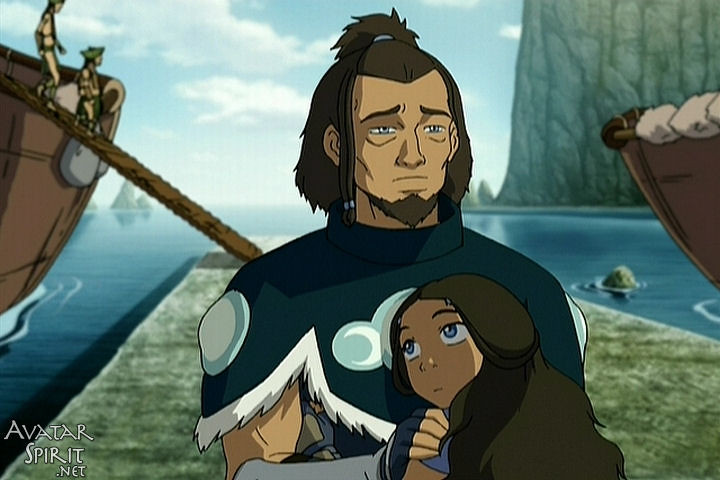In this detailed cartoon screenshot from Avatar: The Last Airbender, labeled "avatarspirit.net" in slim white print in the lower-left corner, a central scene features a man and a girl standing near a large body of blue water under a daytime sky dotted with white clouds. The man, with medium-length dark brown hair pulled into a ponytail and adorned with beaded strands in front of his ears, has light brown skin, light-colored eyes, and a pointed brown beard. He wears a navy shawl with white fur trim and blue circular patterns. He is hugging the young girl, who has long, fluffy brown hair parted in the middle, light-colored eyes, and light brown skin. 

In the background, there are cliffs on the right side and distant ones in the water. On both sides of the pair are ships; the left one is brown with a wooden plank extending to the shore, allowing what appear to be pirate-like sailors in traditional outfits to disembark. On the far right, the prow of another ship is visible, with bags of produce attached to its side.